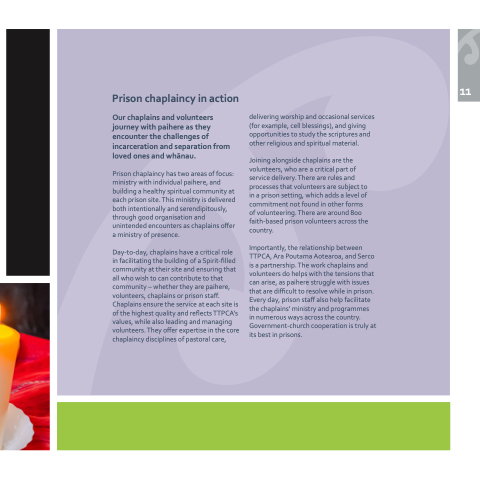The image depicts a page from a book or small magazine, with a violet background and a lime green border at the bottom. The text, under the heading "Prison Chaplaincy in Action," describes the efforts of chaplains and volunteers as they journey with "paihere" (inmates) through the challenges of incarceration and separation from their "whānau" (families). The prison chaplaincy program focuses on two main areas: providing ministry to individual inmates and building a healthy spiritual community at each prison site. This ministry is delivered both intentionally and serendipitously, through organized efforts and unintended encounters, as chaplains offer a presence that supports the spiritual well-being of those in prison. The remaining text, spread over four more paragraphs, further elaborates on the ministry's impact and approach.